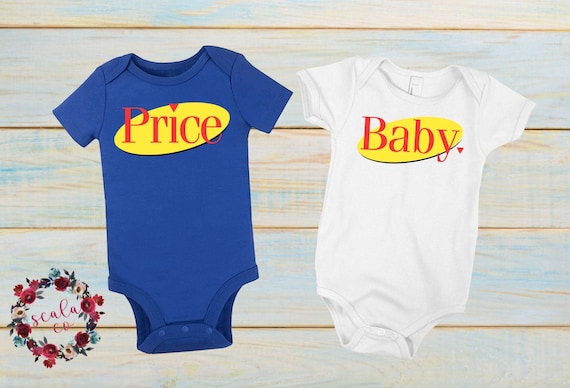The image features two baby onesies laid against a background of light wooden planks, characterized by white with streaks of very light brown and hints of light blue. The onesie on the left is blue and bears an off-center yellow oval on its chest, with red lettering that reads "Price," reminiscent of the Seinfeld logo. The right onesie is white with a similar yellow oval featuring red lettering that reads "Baby," also drawing inspiration from the Seinfeld logo. Positioned at the bottom left of the image is a floral wreath logo composed of red, white, and blue roses. Inside the wreath, in red script, it reads "Scala Co."